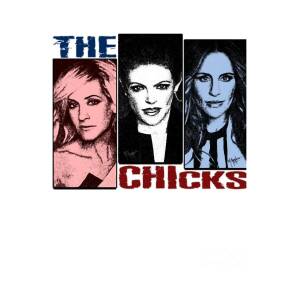The image appears to be a cover for a music CD by the band The Chicks, formerly known as The Dixie Chicks. Centered in a larger white background, three vertical rectangles stand side-by-side, each containing a stylized image of a woman. The background for each rectangle is black, with the woman on the left having a red tone and a slight leftward gaze, the woman in the middle depicted in white facing forward, and the woman on the right presented in blue with long hair and also looking directly at the viewer. In the upper left-hand corner of the image, there is text in blue capital letters reading "THE," and in the bottom right-hand corner, red capital letters spell out "CHICKS." This clean and minimalist design uses the colors red, white, and blue, possibly reflecting a thematic choice related to the band's American roots.